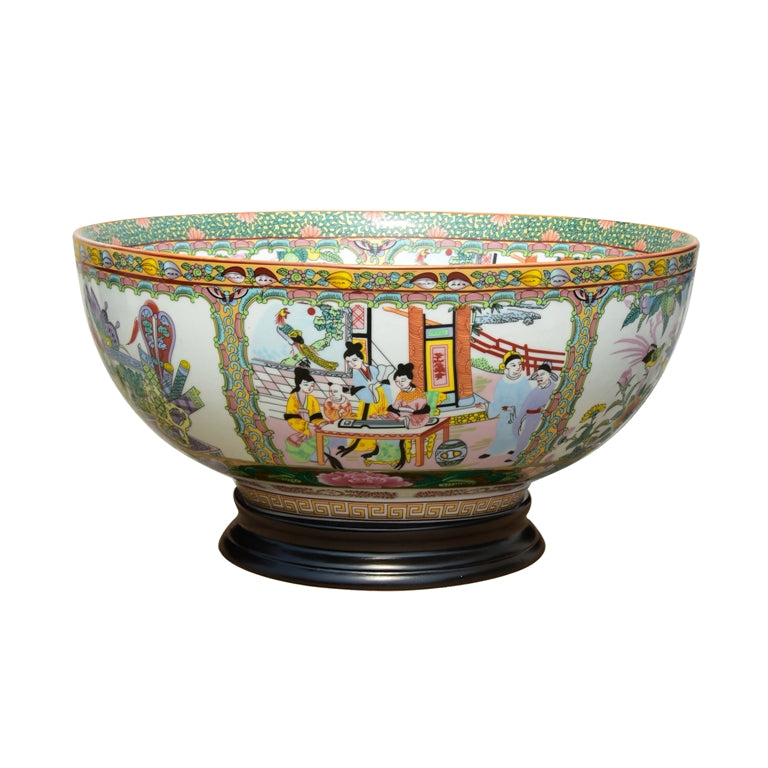This is a detailed product photograph showcasing an exquisite Asian art-style glass bowl with a wooden foot. The dark brown wooden base is about half an inch thick, providing a sturdy foundation for the vibrant bowl. The bowl itself is a canvas of intricate artistry, adorned with scenes of an Asian family dining together, detailed with colorful characters wearing traditional attire in shades of blue, green, and other vibrant colors. Surrounding the family, there are numerous colorful parrots and birds adding to the lively and festive atmosphere of the scene depicted.

The lip of the bowl features elaborate patterns, highlighted with a yellow band on the outside that showcases various fruits and vegetables. The inner lip contrasts this with a green background decorated with delicate cherry blossoms encircling the perimeter. Every inch of the bowl is meticulously painted, creating a rich tapestry of traditional Asian culture and nature. The intricate details and the vivid palette of pinks, greens, yellows, and whites make this bowl a captivating piece of art.